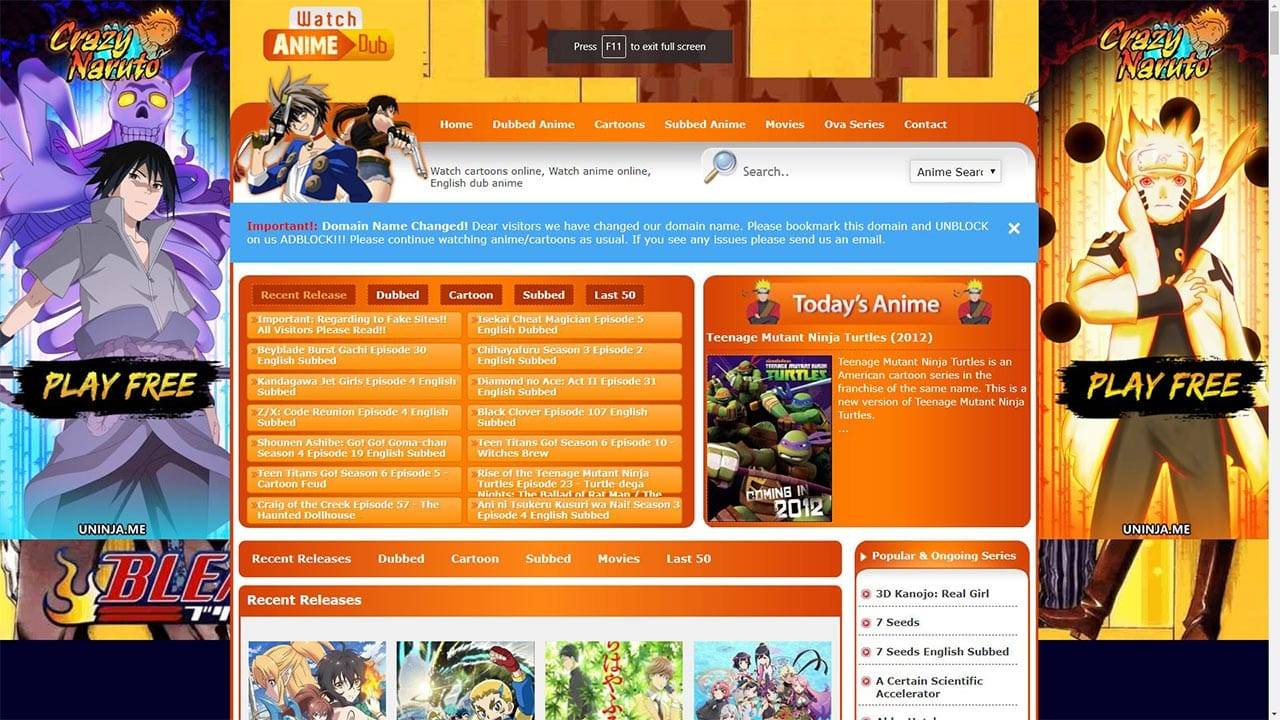The image depicts a vibrant website dedicated to anime content, prominently featuring the banner "Crazy Naruto" on the left side with an invitation to "play free." At the center, there's a striking cartoon illustration of a character with black hair, accompanied by a monstrous figure with a purple body and yellow eyes looming behind him. The text overlay reads "You, Nia, Me" with "BBL" written underneath in bold red letters against a fiery background. 

The top border of the site displays "Watch anime dub," and an instruction to "press F11 to set full screen." Below this, an orange navigation bar features various clickable categories. To the right, there's a search bar labeled "Anime Search" for user convenience. A blue bar spans across the page, though the text within it is too small to discern.

Further down, an orange section with gold text highlights today's anime, featuring the cover image of "Teenage Mutant Ninja Turtles" from the 2012 series. Below this section, thumbnails of four recent releases are visible, though they are partially cut off, only revealing the tops of the images.